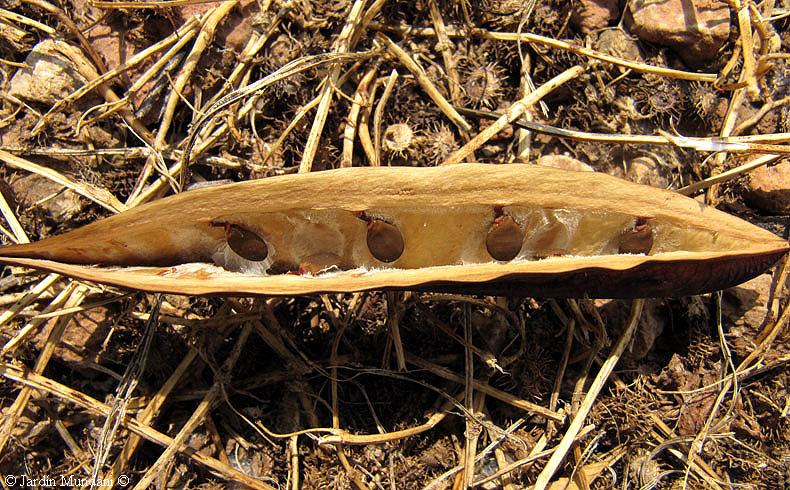This is a horizontally aligned, rectangular photograph depicting a very dry and cracked-open seed pod, possibly from a Moringa plant, resting on a ground covered with dried plants and stems that resemble straw. The scene is predominantly brown with various shades, ranging from light brown, resembling sun-bleached straw, to darker browns that define the exterior of the pod. The pod itself contains a few round, brown seeds nested in small indentations, some of which are surrounded by patches of white. The seeds contrast with the light brown inner membrane of the pod. The background is composed of small sticks, dried grass, and remnants of what once may have been flowers, with occasional accents of rocks in different shades of brown. In the bottom left corner, the image is marked with the copyright text, "Copyright MUNIANI."